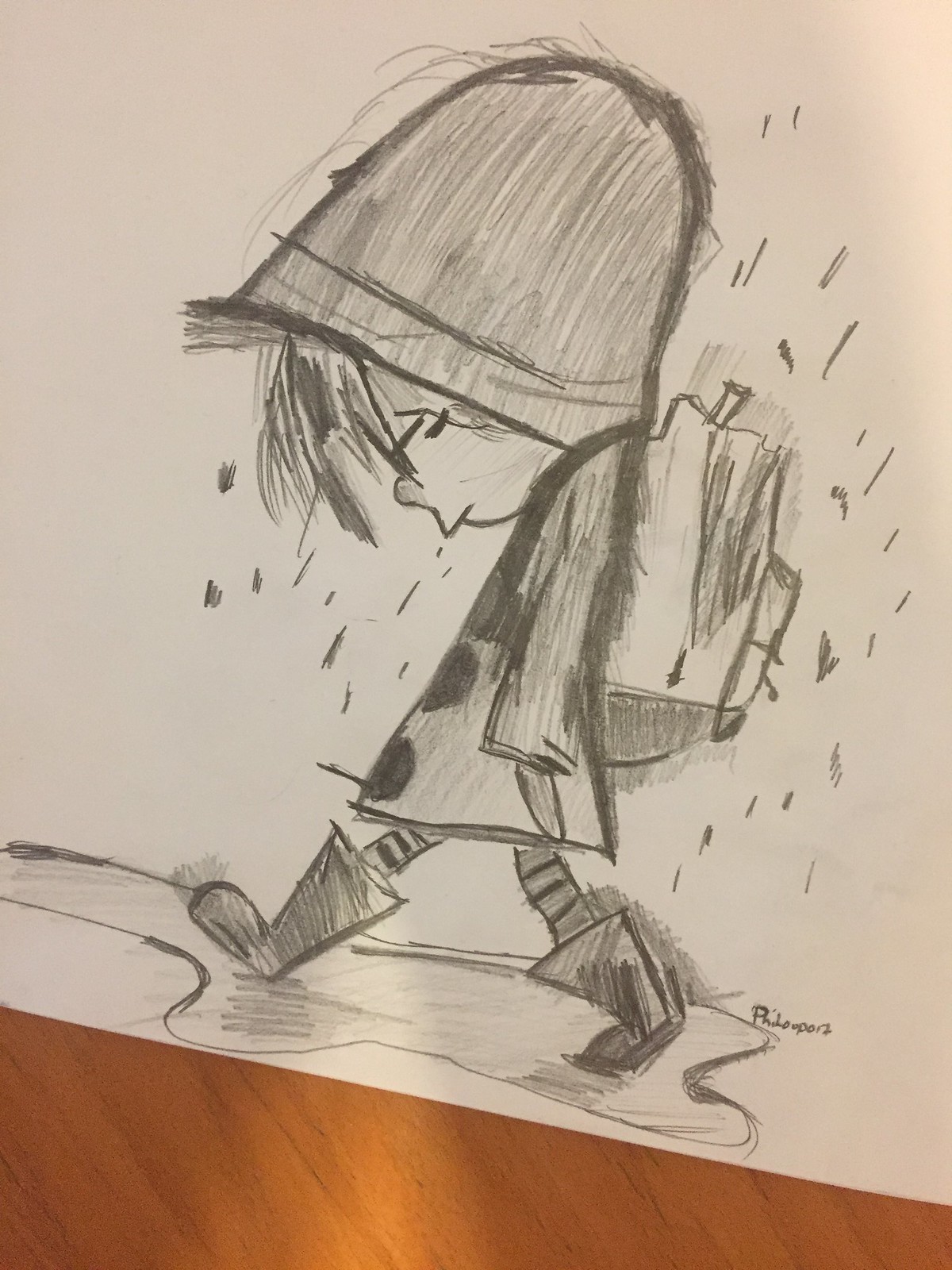This photograph captures a detailed pencil sketch on white artist's paper, lying on a light wooden table, partially visible at the bottom of the image. The sketch depicts a little boy walking in the rain, his head bowed and eyes closed, evoking a sense of sadness. He is dressed in a raincoat with a rounded hood, from which several long strands of hair hang down in front of his face and out the top. He also wears rain boots and striped pants or tights. The boy carries a large backpack on his back as he trudges through a puddle, surrounded by simple pencil-drawn raindrops. The artist’s signature is situated to the right of the puddle, providing a final touch to the melancholic scene.